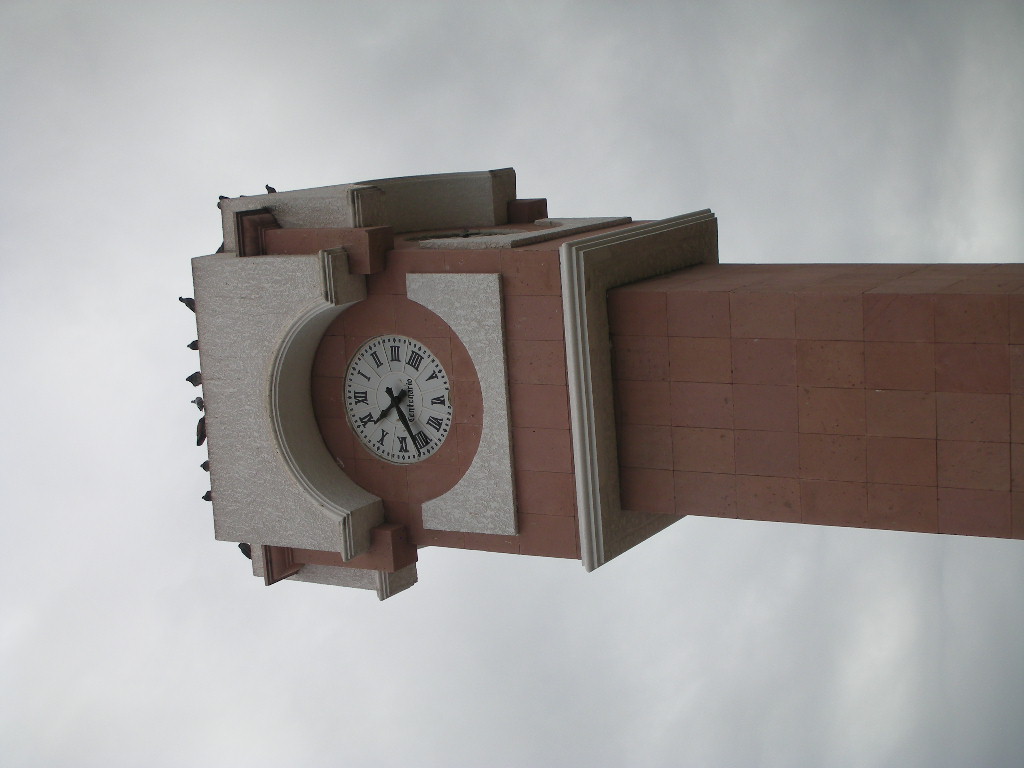The image depicts a clock tower constructed from concrete and red bricks, viewed from a side angle. The prominent clock face, centered within a square base of red bricks, features black Roman numerals from 1 to 12, starting from the left, and meticulously detailed minute dots. The hands of the clock, sharp and arrow-like, indicate the time as 10:40. At the top of the tower, multiple birds, likely pigeons, perch both on the roof and along the sides, adding a lively touch to the scene. The background is dominated by a grey, cloudy sky, suggesting an impending storm. The entire structure exudes a historic and robust aesthetic with its red brick foundation and the grandeur of its concrete clock face.